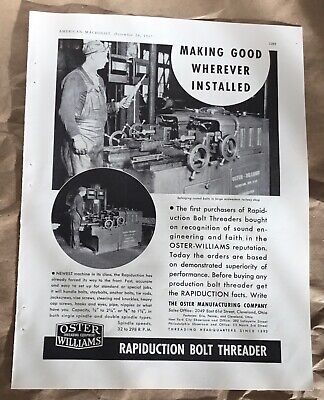This image captures an old advertisement, seemingly from a magazine or a book page, for the Oster Williams Rapidduction Bolt Threader. The page has a white margin and possibly a publication name and page number at the top. The central focus is on two black and white photographs of a man operating a complex machine, possibly a bolt threader.

At the top, a semicircular caption reads, "Making good wherever installed," above the first photograph. This image is a close-up of a man, dressed in overalls, a long shirt, and possibly a hard hat, using the machine.

Below this, intersecting the close-up photo on the left side, is a circular picture offering a clearer, full view of the man and the machine. These images emphasize the operational excellence and design of the machine.

Underneath the circular picture, there is detailed text describing the product. Key phrases include, "The first purchasers of Rapidduction Bolt Threaders bought on recognition of sound engineering and faith in the Oster Williams reputation. Today, the orders are based on demonstrated superiority of performance." It concludes by instructing potential buyers to write to the Oster Manufacturing Company for more information.

At the bottom left, marking the company’s branding, "Oster" is prominently displayed above "Williams" in a distinctive trapezoid shape. To the right of this, a black call-out box spans the width of the page and reads "Rapidduction Bolt Threader," reinforcing the product's identity.